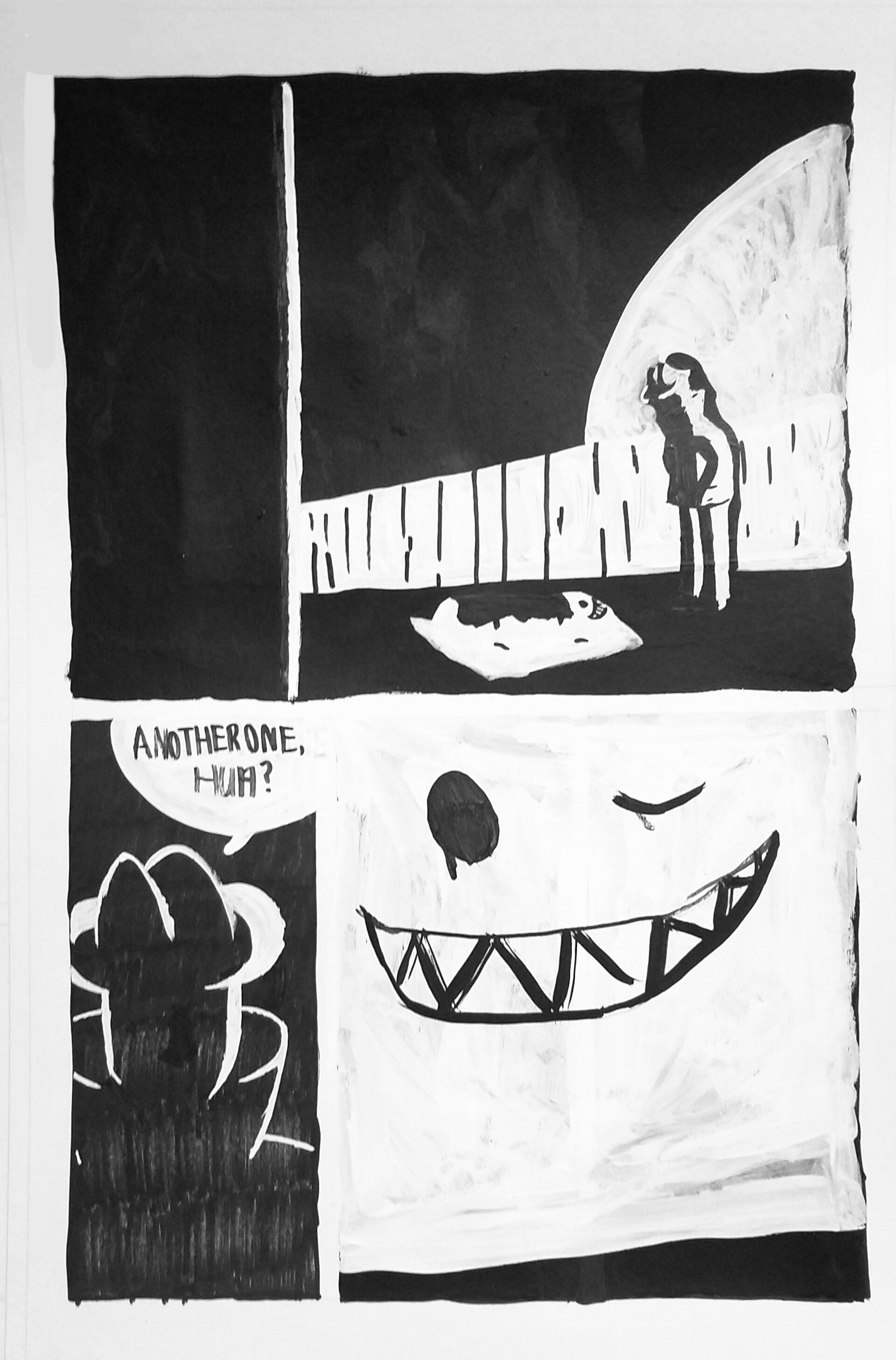This black-and-white artwork, potentially a print or a painting, is structured like a rudimentary comic strip with four distinct panels. The piece is laid out on a tall, narrow sheet of paper and divided into an upper and lower section. Each section is then split into two frames - top left, top right, bottom left, and bottom right.

The top frame features an entirely black background, setting a dark scene. In this panel, a person appears to float or walk in the air, seemingly above a menacing blob with a jagged smiley face, the blob watching them from the ground. This first panel is haunting and establishes a feeling of tension.

In the subsequent panels, the story progresses with more abstract imagery. The second frame might depict the person standing against a fence with the moon in the background, looking down. The third panel includes the only text, where the person seems to say, "Another one, huh?". This dialogue hints at a reflective or resigned tone.

The final panel shows a more abstract face, with one eye winking and the other open, sporting a jagged smile. This image adds to the overarching surreal and enigmatic nature of the artwork. The entire piece appears somewhat unpolished, with a style that suggests it was executed with markers, reflecting a raw, expressive quality meant to convey a deeper message or narrative.